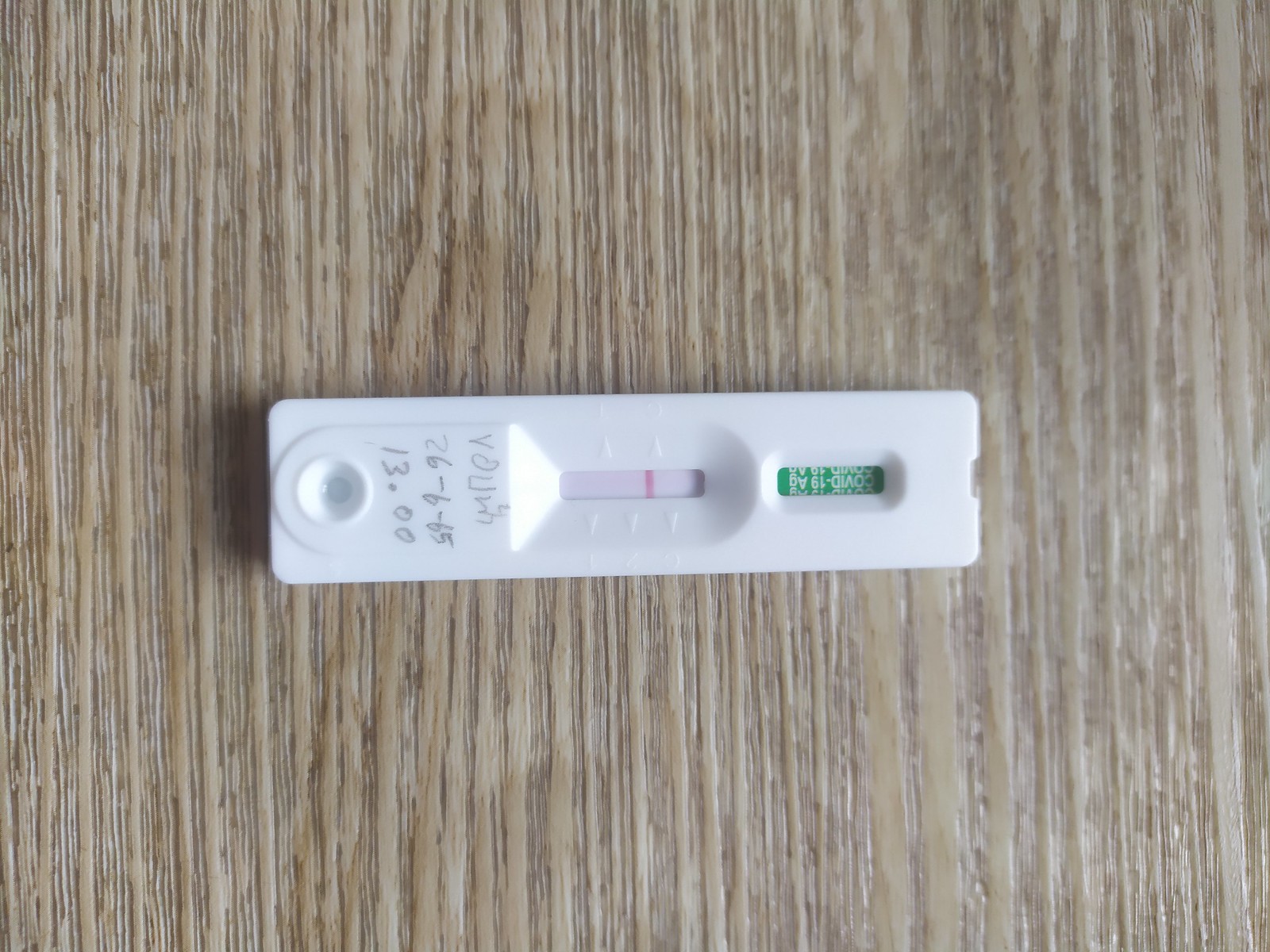The image depicts a brightly lit photograph set against a light-colored wooden background with reflective tones. The focal point of the photo is a rectangular white plastic COVID-19 test, prominently displaying "COVID-19" in green lettering. Designed for sample dripping, the plastic test features a dedicated spot for the liquid sample. The test is a PCR type, marked with arrows and currently showing one red line, indicating a negative result. If it were positive, two red lines would be visible. The round part of the test still contains some liquid. Additionally, there is some scribbled writing in pencil on the test, spelling out "V-O-U-H". Below the writing, the birth date "6-26-65" and the time "13:00" are messily noted, suggesting when the test was administered.